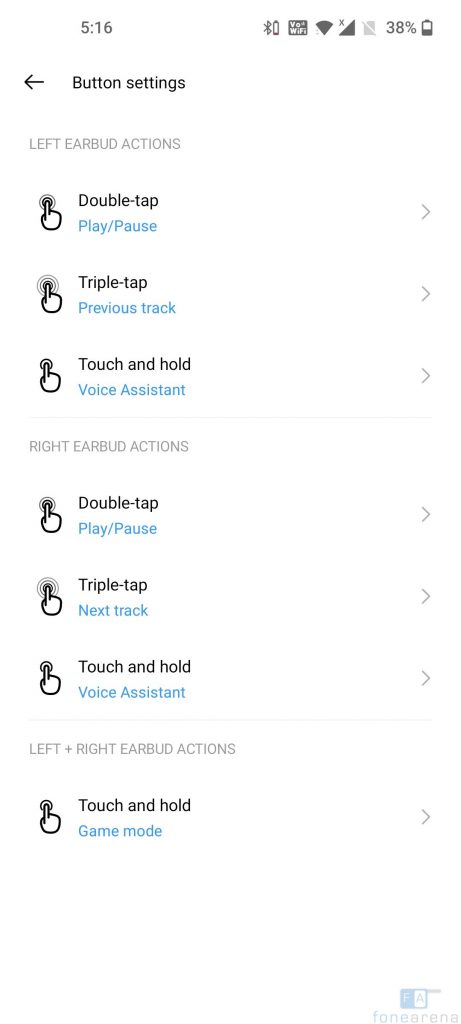The image displays a screenshot with a white background, captured from a smartphone at 5:16 AM. The status bar shows a fully connected Wi-Fi signal and a battery life at 38%. Below the status bar, on the left side of the screen, there is a back arrow labeled "Button settings."

Under this, the section titled "Left Earbud Actions" features a list with corresponding icons on the left, resembling earbuds, and right-pointing arrows on the right. The list includes:
- Double tap: Play/Pause
- Triple tap: Previous Track
- Touch and hold: Voice Assistant

Following this, another section is labeled "Right Earbud Actions," containing similar information with slight variations:
- Double tap: Play/Pause
- Triple tap: Next Track
- Touch and hold: Voice Assistant

A final section titled "Left & Right Earbud Action" indicates a combined functionality:
- Touch and hold: Game Mode